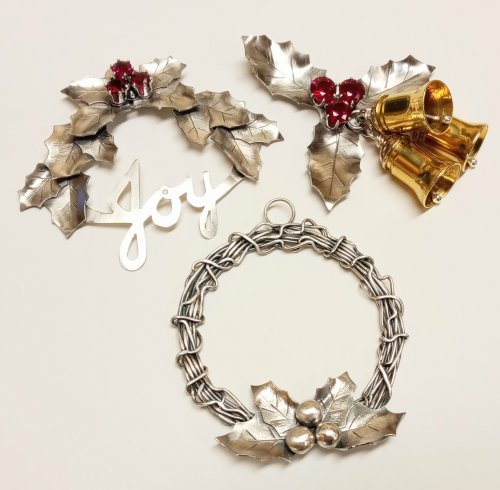The image depicts a Christmas card featuring three intricate pieces of holiday-themed jewelry, all set against an off-white background. Each piece prominently incorporates holly or mistletoe motifs, emphasizing a festive aesthetic. 

In the top left corner, there is a silver brooch with holly leaves cascading down either side from a central red jewel, possibly a ruby. The word "Joy," crafted from silver metal, spans the width of the holly leaves, enhancing the holiday sentiment.

In the top right corner, another brooch showcases three silver leaves, likely holly or mistletoe, each converging at a cluster of three red jewels. Dangling from these leaves are three small, golden bells that add a touch of whimsy and festivity.

Dominating the bottom third of the image is a circular ornament made of braided silver. It features a tiny loop at the top, suggesting it could be hung on a tree. At the bottom of the circle is a cluster of four silver holly leaves centered around three silver berries, continuing the cohesive color theme.

All pieces reflect a harmonious blend of silver and gold hues, with pops of red from the various jewels, creating an elegant and festive presentation suitable for a holiday card.